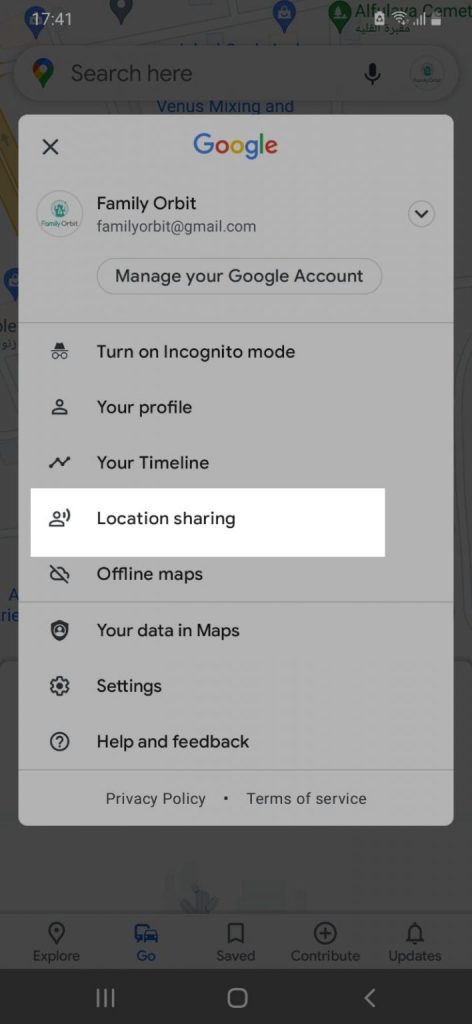This image is a screenshot from a smartphone, captured at 17:41, as displayed in the top left corner. In the upper right-hand corner, the Wi-Fi, service, and battery icons are visible. The background features Google Maps with the familiar "Search here" bar at the top and a row of icons at the bottom.

Superimposed on this background is a Google Account alert. At the top of this alert, the word "Google" is prominently displayed, followed by a menu icon. Below, the account name 'Family Orbit' (familyorbit@gmail.com) is shown along with its profile picture. Beneath this, there is a button labeled "Manage your Google Account."

The menu options listed are: Turn on Incognito Mode, Your Profile, Your Timeline, Location Sharing, Offline Maps, Your Data in Maps, Settings, and Help & Feedback. The "Location Sharing" option is currently selected, highlighting this feature.

At the bottom of the Google Maps interface, the icons from left to right are: Explore, Go, Saved, Contribute, and Updates, each represented by its respective pictorial symbol.